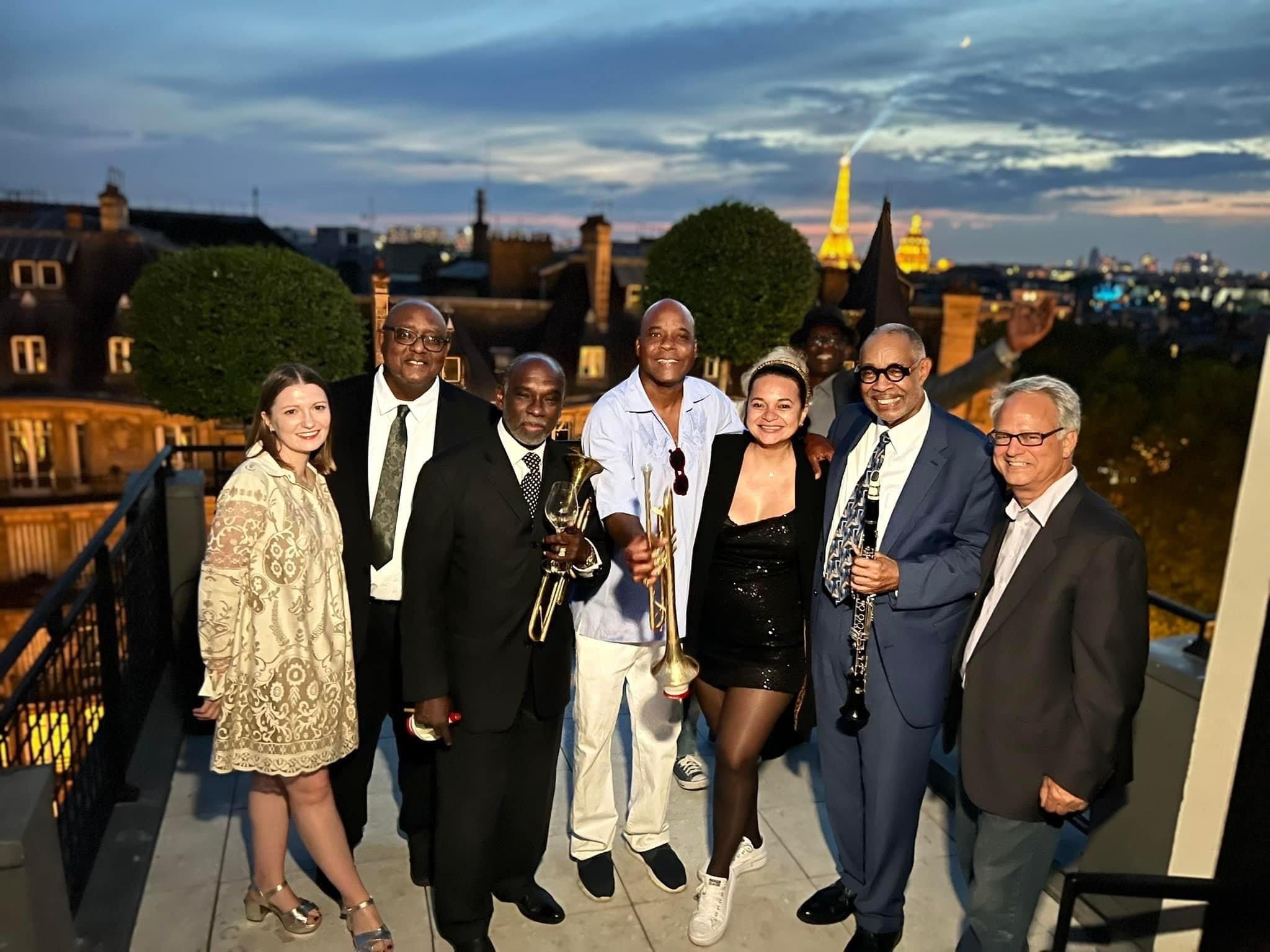In this nighttime photograph, a diverse group of seven people—mostly of African descent and one white woman—are gathered on a balcony or rooftop, posing and smiling warmly at the camera. The group comprises five men and two women. All the men are dressed in suits with white collared shirts, and three of them wear glasses. The women add to the elegance, with one in a loose-fitting, gold print shift and the other in a sequined black short dress paired with a jacket. Some members of the group appear to be musicians, holding instruments: two men are holding trumpets, and one is holding a clarinet. Two others are holding glasses of wine, adding a celebratory touch to the scene. The backdrop features the lit-up Eiffel Tower towering above the city's skyline, hinting at the end of twilight with city lights beginning to twinkle. The sky is cloudy, suggesting that the sun has just set. This cohesive group, seemingly a band, exudes a sense of joy and camaraderie.